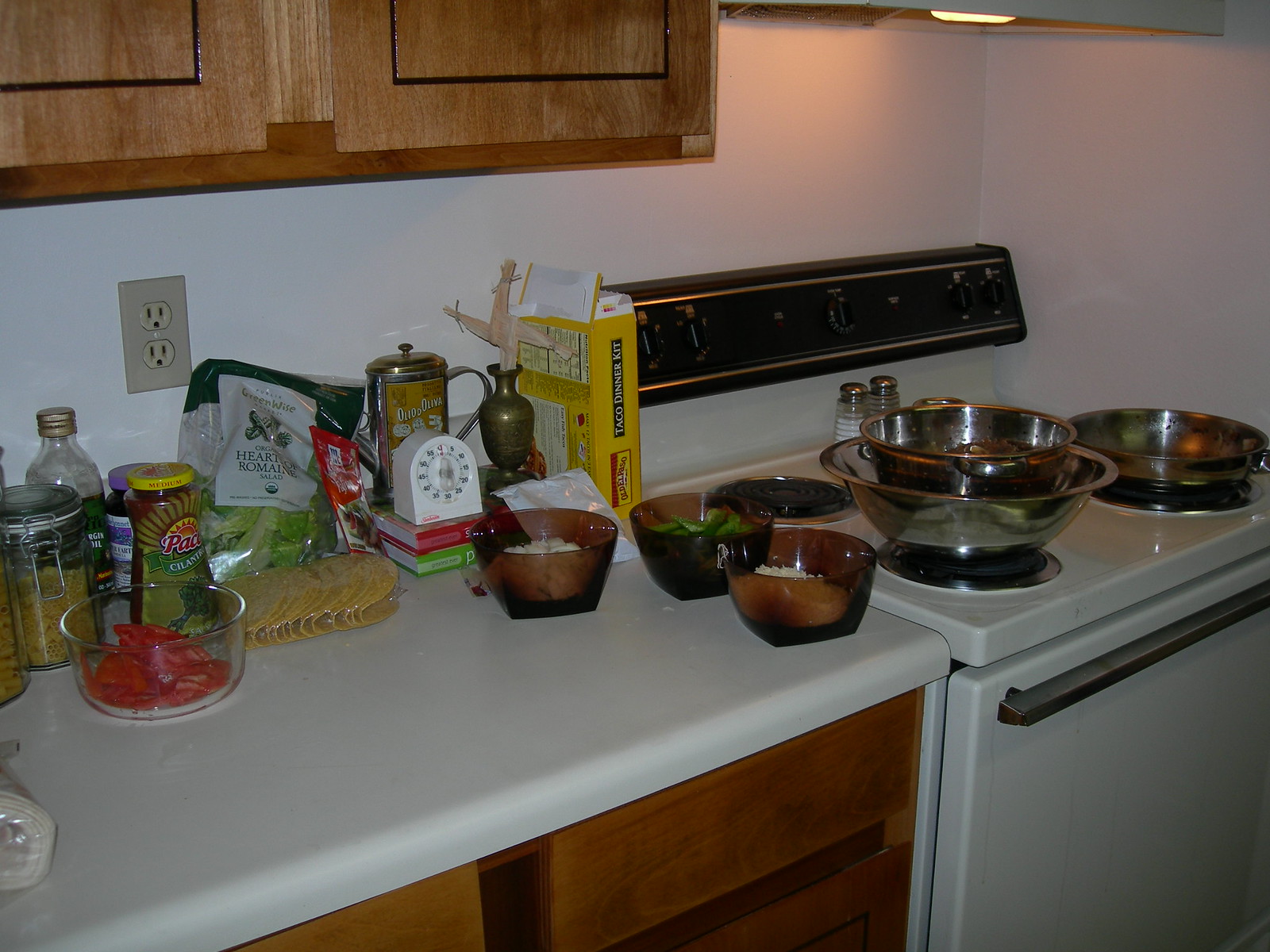The photo captures a bustling kitchen scene, with a countertop and a vintage white gas stove taking center stage. The countertop is cluttered with a variety of cooking ingredients and utensils, indicative of a meal in progress. Visible items include bags of salad greens, ripe tomatoes, a bottle of cooking oil, tortillas, green peppers, onions, and possibly some shredded cheese. Additional condiments, jars, and boxes are scattered around, alongside a timer and several cooking books, signifying an active cooking environment. Metal bowls and a metal pan are placed on the stove, whose light is turned on, illuminating the area. The old-fashioned stove features classic knobs for adjusting the heat levels. An electric plug on the wall is also observed, ready for any additional appliances. Though no person is visible in the photograph, the scene clearly shows the kitchen is halfway through preparing a meal.